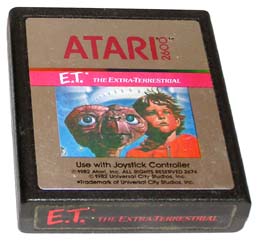This is a detailed photograph of an Atari 2600 game cartridge for the video game "E.T. the Extra-Terrestrial." The cartridge itself is black with a tan label affixed to its front. At the very top of this label, in bold red letters, it says "Atari 2600." Directly below, a lighter red horizontal banner bears the white text, "E.T. the Extra-Terrestrial." Underneath this banner is an artistic depiction from the iconic movie: E.T., the creature with a long neck and large eyes, standing next to a little boy with sandy blonde hair, blue eyes, and wearing an orange or red jacket. Their faces are close together, almost touching. Below this image, in black letters, the text reads, "Use with Joystick Controller" alongside some additional, less legible text and copyright information stating, "All rights reserved. Universal City Studios Incorporated." Along the bottom edge of the cartridge, the title "E.T. the Extra-Terrestrial" is repeated in red letters against the black background of the cartridge.